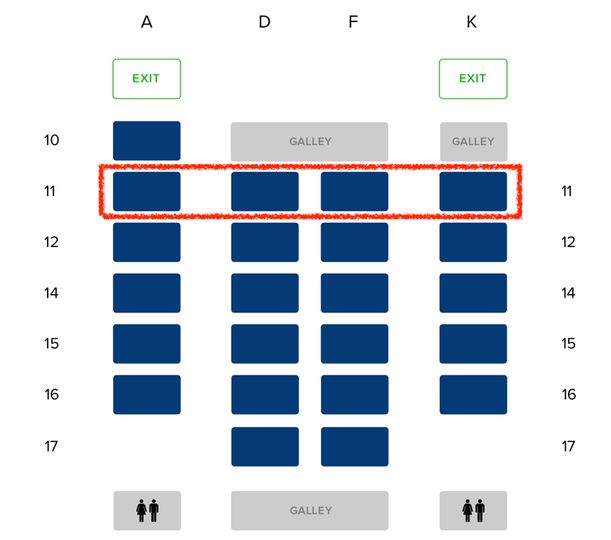This square seating layout diagram on a white background features clearly marked components without a defining border. At the top, four columns labeled A, D, F, and K in black text are present. Directly below these columns, green boxes with the word "Exit" in green text are seen.

On the left-hand side of the image, the rows are labeled with numbers 10, 11, 12, 14, 15, 16, and 17 in sequence. Mirroring these on the right side are the same row numbers. Starting from row 10, a blue box marked "Galley" spans across the width of columns A and D. Adjacent to this galley, another identically sized blue rectangle is placed within column F and K.

The next row consists of four blue, landscape-oriented rectangles with a red box drawn around them. Following this, row 14 has a similar configuration with four blue rectangles, but it is not highlighted. Rows 15 and 16 also have four blue rectangles each.

In row 17, only two blue rectangles are centered within the layout. Below these rectangles, another "Galley" is marked in gray, matching the width of the two blue rectangles above it. At the very bottom of the image, on either side of the gray galley, restroom indicators are situated. These indicators feature universally recognized symbols for women and men.